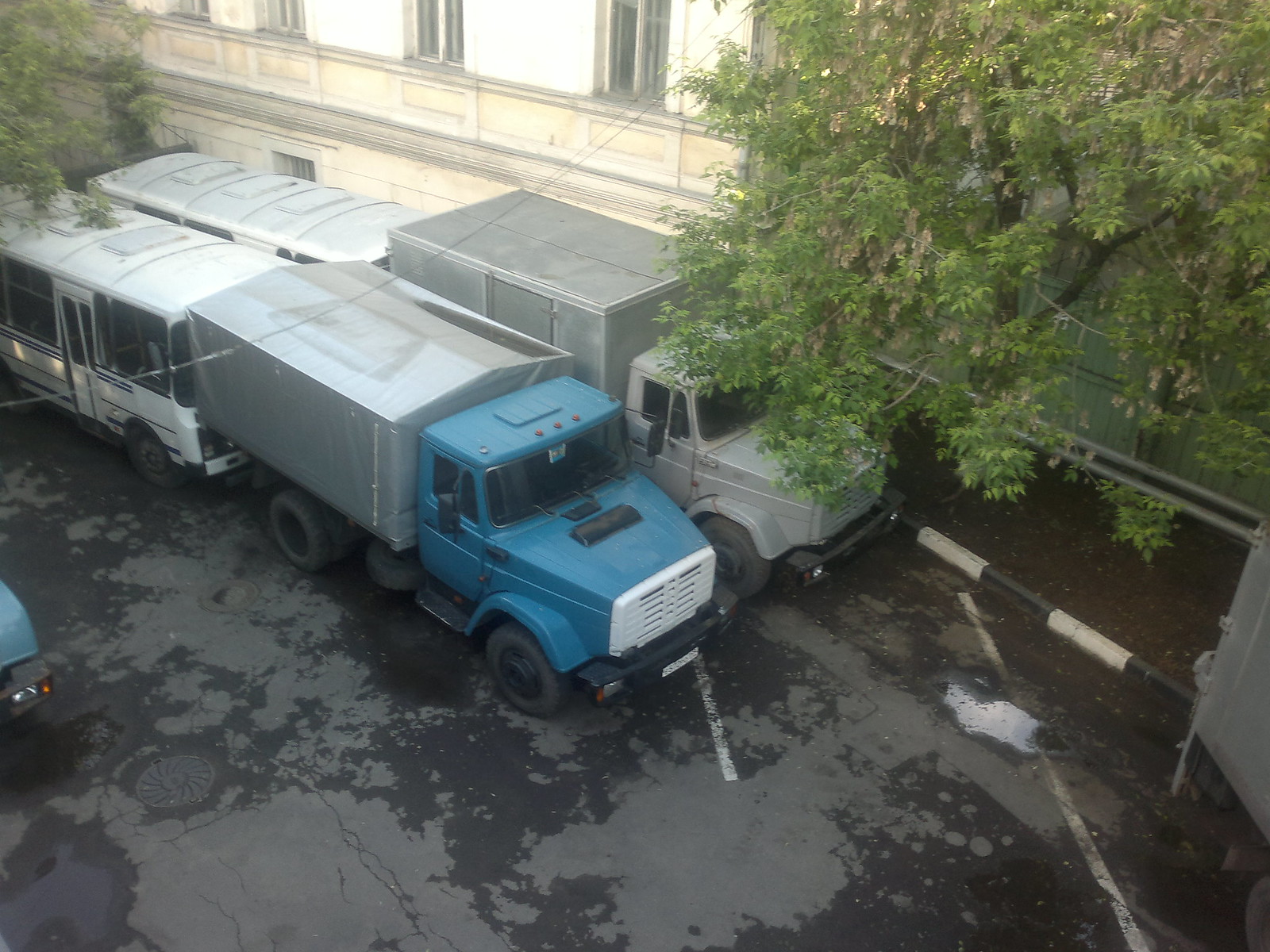In this detailed image, two large trucks are closely backed up against two identical white buses, sandwiched together on a splotchy black and gray pavement. The truck on the right features a gray cab with black windows, black rearview mirrors, a black bumper, black tires, and a gray box on the back with a door. Adjacent to it, the truck on the left mirrors the structure of the right truck but has a distinctive blue cab, white grille, and similarly equipped gray box with a slight peaked roof. Directly behind each truck, the white buses have lines running across their roofs with rectangular indentations between each line. The scene is framed by trees on either side and a two-story building with visible white windows in the background. Additionally, the lower right corner reveals a bar to a gate, hinting at access to an underground parking area.